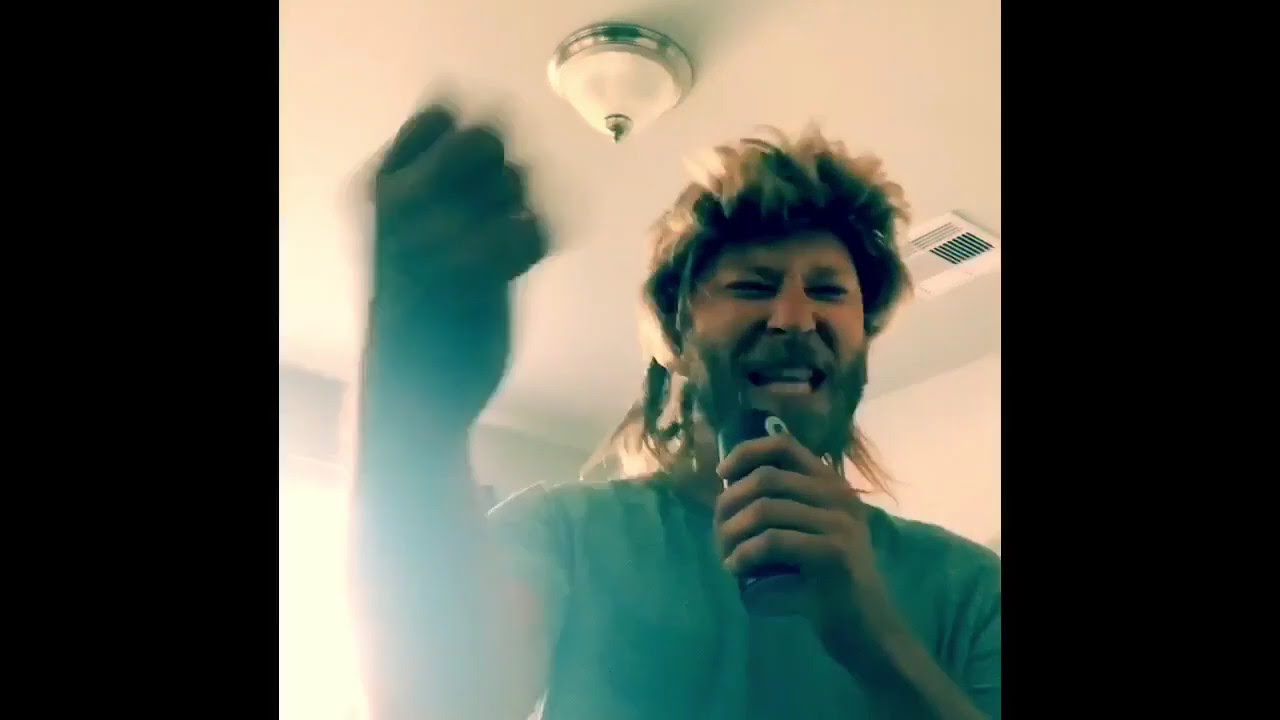This vibrant photo captures a middle-aged man, positioned under a white ceiling with a light fixture and a vent to the right of his head. Sporting a classic 80s mullet—a blend of brown hair with blonde-dyed ends—his voluminous hairstyle is disheveled yet piled high, with visible strands cascading down his neck. 

The man’s expression is dynamic and energetic, with eyes scrunched tightly shut and mouth wide open, revealing all his teeth, as if he's in the midst of an impassioned yell or song. His face is adorned with gray stubble, adding a rugged texture to his intense demeanor.

He's dressed in a medium green t-shirt, and his right fist, slightly blurred and clenched, is raised in an animated gesture towards us, implying vigorous movement. In his left hand, held up to his mouth, is a makeshift microphone—a black cube that he's actively singing or shouting into.

The photo is taken from a lower angle, enhancing the man's presence and emphasizing his energetic performance in this simple, white-walled room.